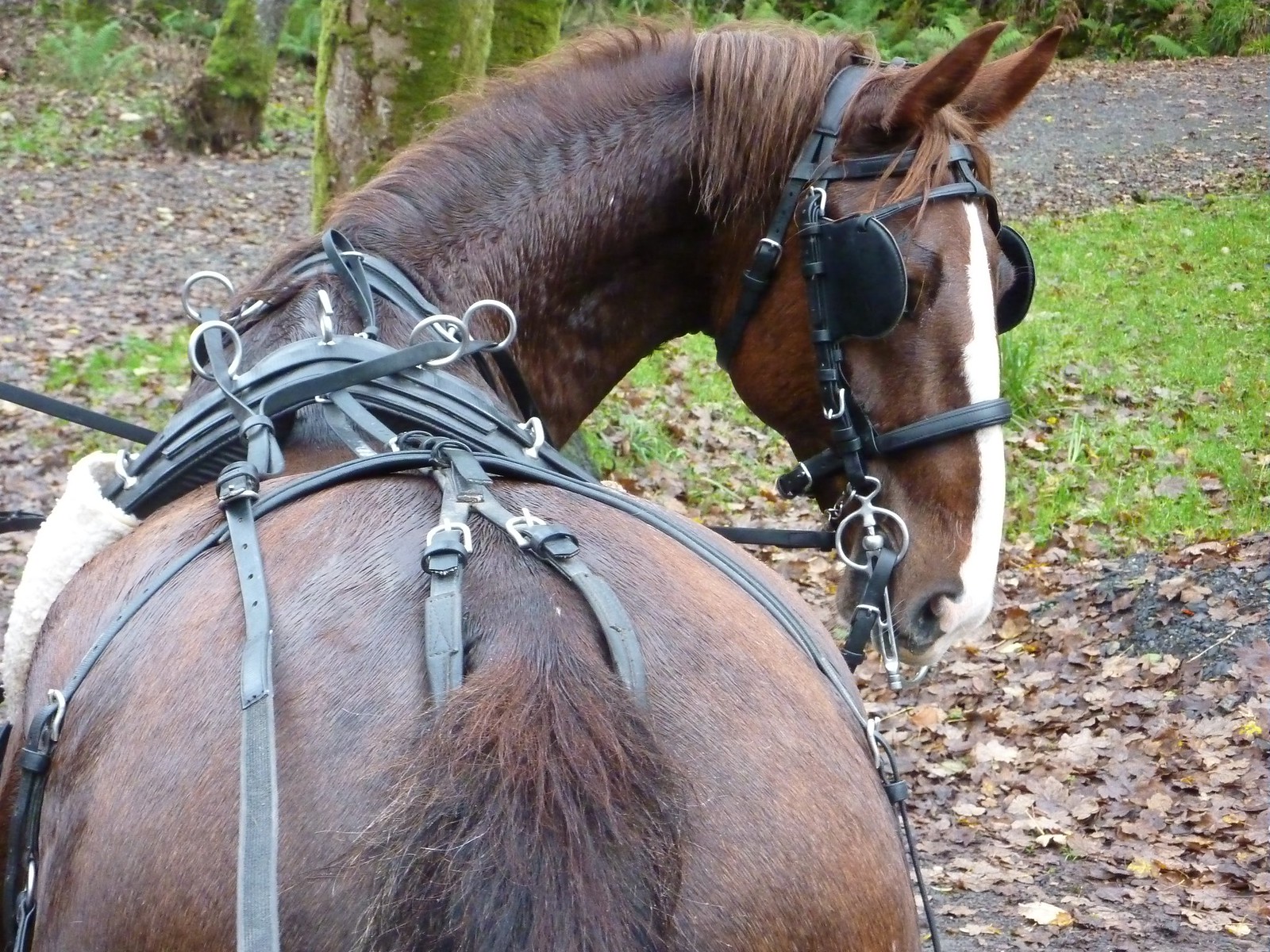In this color landscape photograph, a majestic brown horse stands against a backdrop of fallen autumn leaves and greenery, with trees adorned in moss. Captured from behind, the horse's elegant neck arches in a C-curve as it turns its head almost fully to the right, staring back at the photographer with a keen, focused gaze. The horse, a beautiful chestnut brown with a dark mane and tail, features a distinctive long white stripe that stretches from its nose up to its ears. 

Adorned in a full set of riding gear, the horse wears a black saddle fastened securely around its belly and hooked underneath its tail, featuring silver accents and a handhold near the top. Straps run from the bridle on its head to the saddle, while blinders beside its eyes help keep its attention forward. Although no legs are visible in the image, the horse appears well-prepared for riding with reins, bridle, and stirrups in place. The seasonal setting, likely fall, enhances the scene with lush green grass peeking through a blanket of earthy brown leaves.